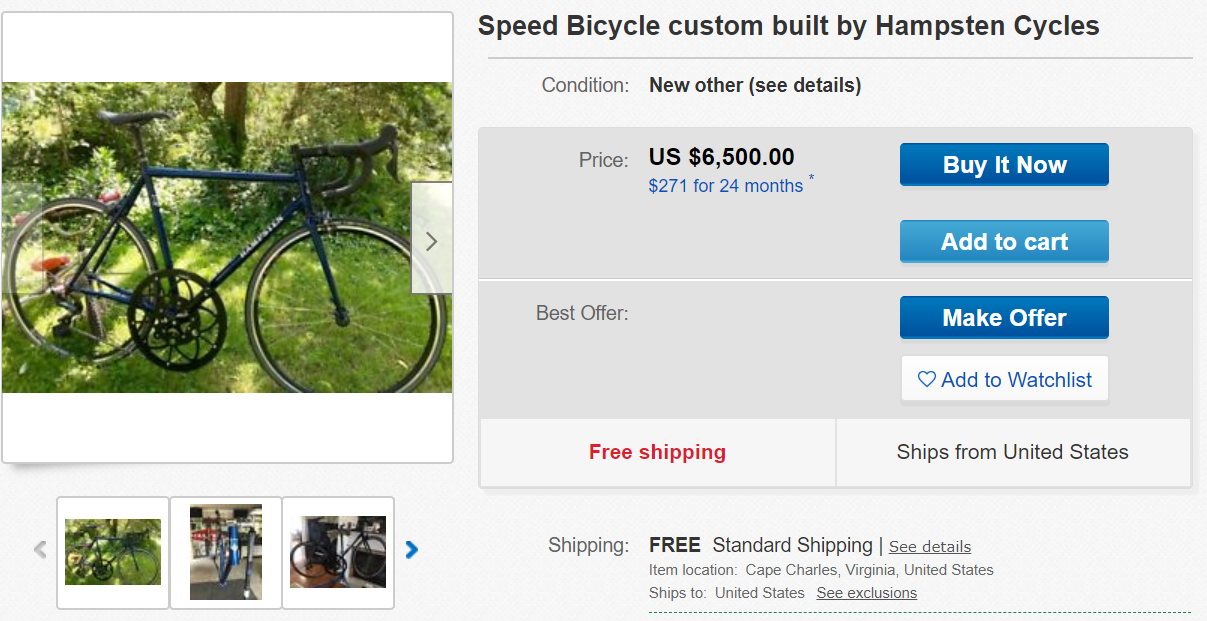### Detailed Caption for Product Image

This rectangular landscape image showcases a bicycle being sold online, divided into two primary sections: the product display on the left and the description with purchasing options on the right.

#### Left Side (Approximately 35% of the Image):
- **Main Bicycle Image**: At the top left, a nearly square photograph features the bicycle positioned outdoors on lush green grass with a backdrop of trees. The white margins at the top and bottom frame the image neatly. The bicycle itself is a sleek, black, tall, and thin model with curved racing handles and multiple gears, standing upright on its kickstand, facing right.
- **Additional Bicycle Thumbnails**: Beneath the main image is a horizontal strip containing three small thumbnail pictures of the same bicycle. These are difficult to see in detail but can be scrolled through using the left and right arrows on either side of the strip.

#### Right Side (Approximately 65% of the Image):
- **Product Title and Description**: At the top, bold black text reads, "Speed Bicycle, custom built by Hampstead Cycles," underlined by a gray line that spans the width of this section. Below it, indented slightly, the condition is noted as "New, Other (See Details)" in darker gray text.
- **Price and Payment Options**:
  - Underneath a darker gray background strip, aligned vertically with the above text, "Price:" is stated in bold black, indicating the cost as "US $6,500.00."
  - Below the price, blue text outlines a payment plan: "$271 for 24 months," with a small asterisk next to "months."
- **Action Buttons**:
  - Two rectangular, landscape-oriented buttons are positioned here:
    - The top button in darker blue with white text reads, "Buy It Now."
    - The bottom button in a lighter blue with white text says, "Add to Cart."
- **Best Offer Section**: Separated by a white line, another dark gray box on the left hosts the text "Best Offer:" with no content next to it. To the right, two additional buttons:
  - "Make Offer" in dark blue, identical to "Buy It Now."
  - "Add to Watchlist" with a white background, blue text, and a blue heart symbol.
- **Shipping Information**:
  - Beneath the gray boxes, two side-by-side white boxes offer:
    - "Free Shipping" in red text on the left.
    - "Ships from United States" in black text on the right.
  - Further down, the shipping details include:
    - "Shipping: Free," followed by "Standard Shipping | See Details," the latter underlined.
    - Item location is listed as "Cape Charles, Virginia, United States."
    - "Ships to: United States | See Exclusions," the exclusions text underlined.

This comprehensive layout effectively combines visual displays of the product with detailed purchasing information, ensuring potential buyers have a clear understanding of the bicycle and its sales details.